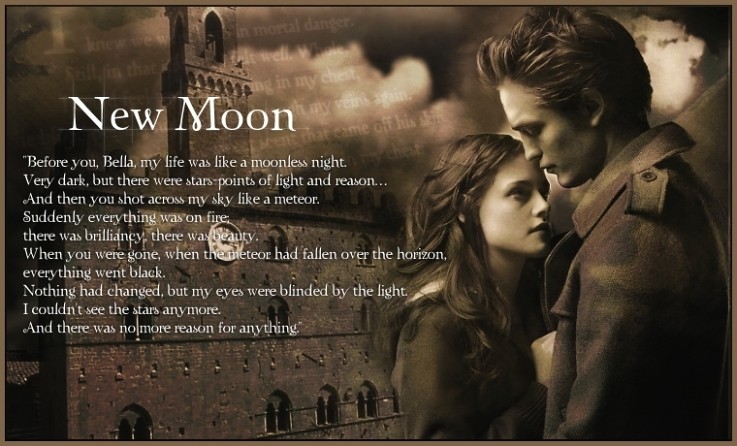The image depicts a movie poster for the Twilight franchise, specifically for the film "New Moon." Dominating the poster, on the left side, is a poignant quote: "Before you, Bella, my life was like a moonless night. Very dark, but there were stars—points of light and reason. And then you shot across my sky like a meteor. Suddenly everything was on fire; there was brilliancy, there was beauty. When you were gone, the meteor had fallen over the horizon. Everything went black. Nothing had changed, but my eyes were blinded by the light. I couldn't see the stars anymore, and there was no more reason for anything." This text is superimposed over an image of an old church.

On the right side of the poster, the scene depicts two main characters: a man with medium-length hair, slicked back, wearing a heavy coat, and looking downward with his eyes closed, and a young woman standing close to him, looking up. The characters are likely meant to represent Edward Cullen and Bella Swan, the central figures in the Twilight series. The poster is rendered in a palette of black, white, various shades of gray, tan, and brown, contributing to its somber and reflective mood. The entire image is consumed by the poster, indicating its importance in setting the tone and theme of the film.